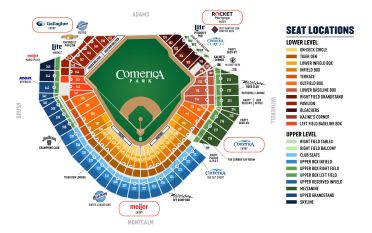The image is a detailed seating chart for Comerica Park, prominently labeled at the top against a green backdrop representing the sports field. The chart clearly outlines a baseball diamond, complete with a pitcher's mound. Surrounding the field are color-coded seating areas, ranging from blue to orange to red to green, each representing different sections of the stadium. 

On the far right of the image, a color key column provides context for the seating categories. Despite being fairly blurry, some text is decipherable. The column headings include "Seat Locations," split between "Lower Level" and "Upper Level." 

The "Lower Level" lists twelve distinct seating sections, primarily shaded in orange, yellow, and brown hues. One identifiable term within this section is "bleachers," corresponding to a darker color visible in the top right area of the seating map.

Below the lower level details, the "Upper Level" section lists ten additional seating areas, marked mainly in shades of green and blue. These upper-level sections are situated towards the bottom and outer edges of the map, indicating their positions further from the field compared to the lower level.

Though some text remains indistinct, the chart effectively conveys the layout and seating distribution within Comerica Park.